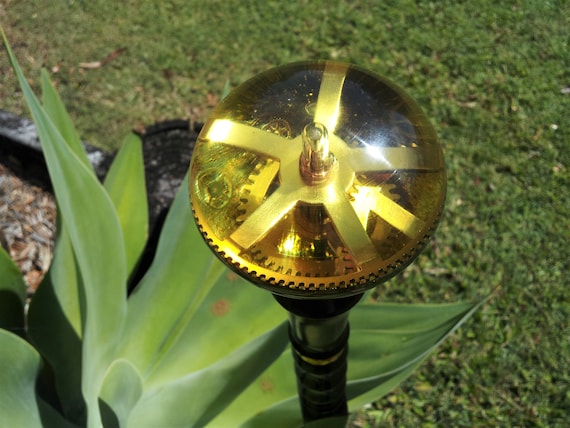The image is a close-up photograph of a mechanical light fixture situated in a yard. The focal point of the image is a spherical, transparent dome of a yellow-gold color at the top, held up by a long black stem extending from the ground. Inside the dome, the intricate inner workings of the light are visible, including several gold-colored gears and what appears to be a filament or LED light in the center. The background is predominantly grass, covering about 60% of the visible area, indicating that the lawn has been recently cut. In the bottom left corner, there is a plant with very large leaves, partially obscuring an area sectioned off with wood chips. The overall perspective of the photo suggests it was taken from an upward angle, capturing the light fixture in a detailed and descriptive manner.